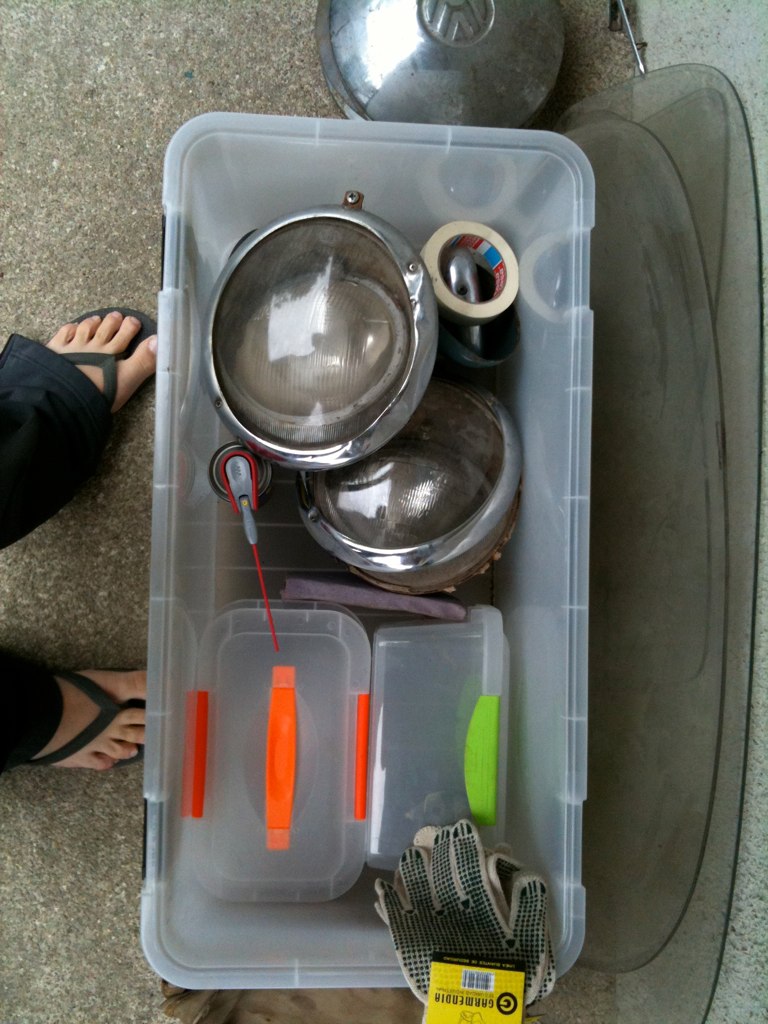This color photograph offers a bird's-eye view of a concrete floor. At the center of the image, a clear plastic storage container reminiscent of a Rubbermaid tote is prominently positioned. The worn concrete floor is also partially bordered by a concrete wall just visible along the far right side. 

To the left, slightly off-center, two feet captured in a V-shaped stance draw attention. Their light-colored skin is adorned with black flip-flop sandals, and they are clad in long, black cotton pants, grounding the scene in everyday practicality.

A round, silver hubcap or car part is conspicuously placed at the top center of the image, adding an industrial touch. 

Inside the plastic container, a variety of objects are carefully placed: two round car headlights encased in silver rims, a roll of masking tape, two smaller clear plastic containers, a pair of black-and-white gardening gloves, and a slender red object with a gray attachment at one end. These items collectively tell a story of meticulous organization, hinting at automotive or DIY activities.